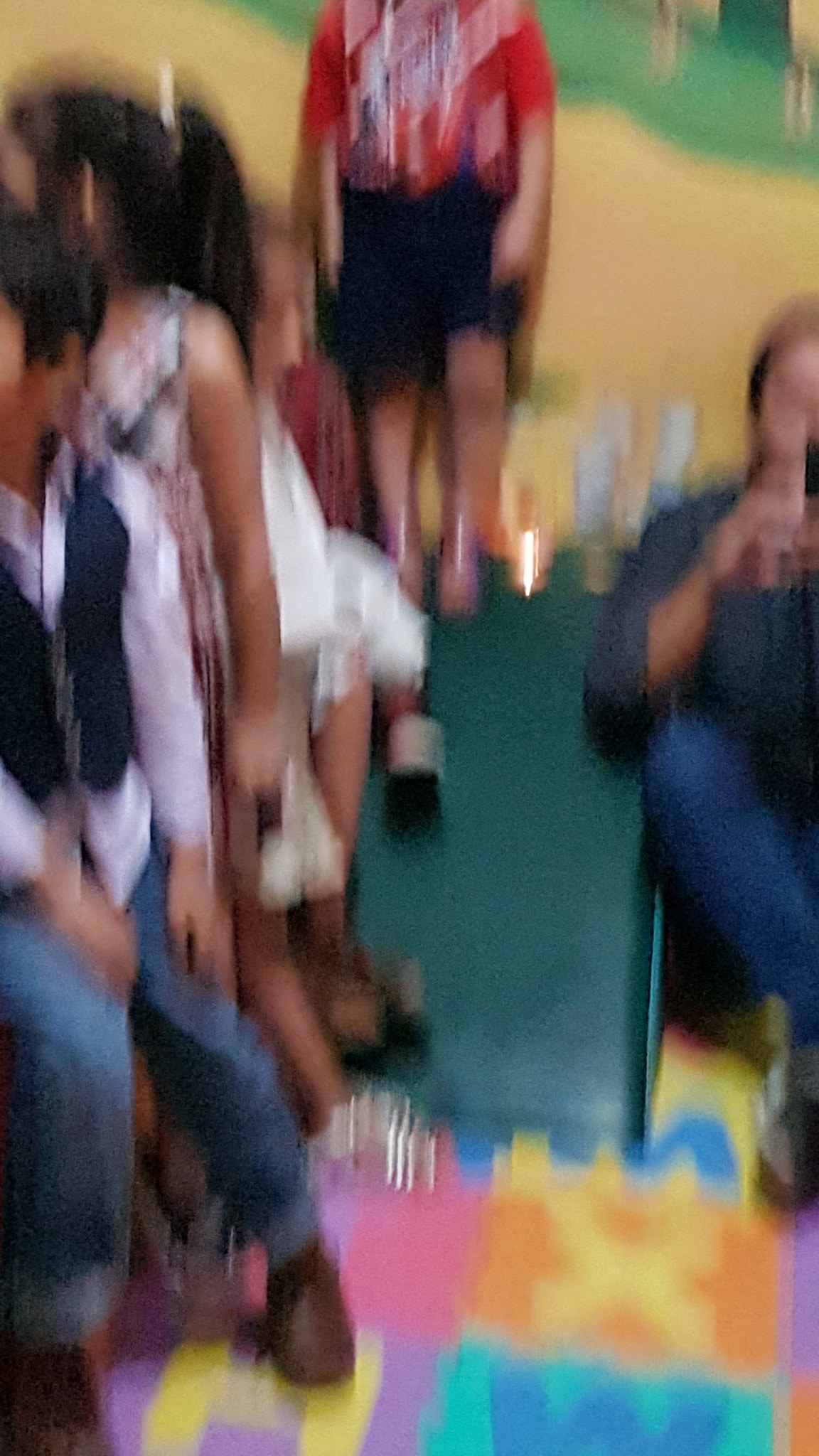The image is a very blurry photograph, seemingly taken in motion, making it difficult to discern specific details clearly. The photo is approximately two and a half to three times taller than it is wide. The scene depicts a vibrant, busy environment, possibly a kindergarten event like a talent show or play, given the presence of colorful elements and children.

At the forefront, there is a multicolored letter mat for kids, typically used in kindergarten, lying on the floor. Positioned on the left side of the mat, several children are seated. Notably, a boy in a dark-colored vest over a white dress shirt, jeans, and brown shoes is visible. Beside him, there is a girl dressed in a white dress with potential pink accents, identifiable by her long brown hair. Another child in a red shirt with graphic design and blue shorts can be seen, though only from the shoulders down.

An adult, possibly a parent, is positioned towards the right side of the image, cut off partially by the edge. This person, who has short hair, wears blue jeans and a blue shirt, and appears to be Caucasian. They sit with their knees up, facing the camera. Additionally, the image reveals a backdrop consisting of a green slide-like object with glasses or bottles lined up on top, complemented by a rippled green and yellow wall section in the upper background.

Overall, despite the blurriness, the image captures a lively and colorful moment, filled with the chaotic charm typical of a children's gathering.